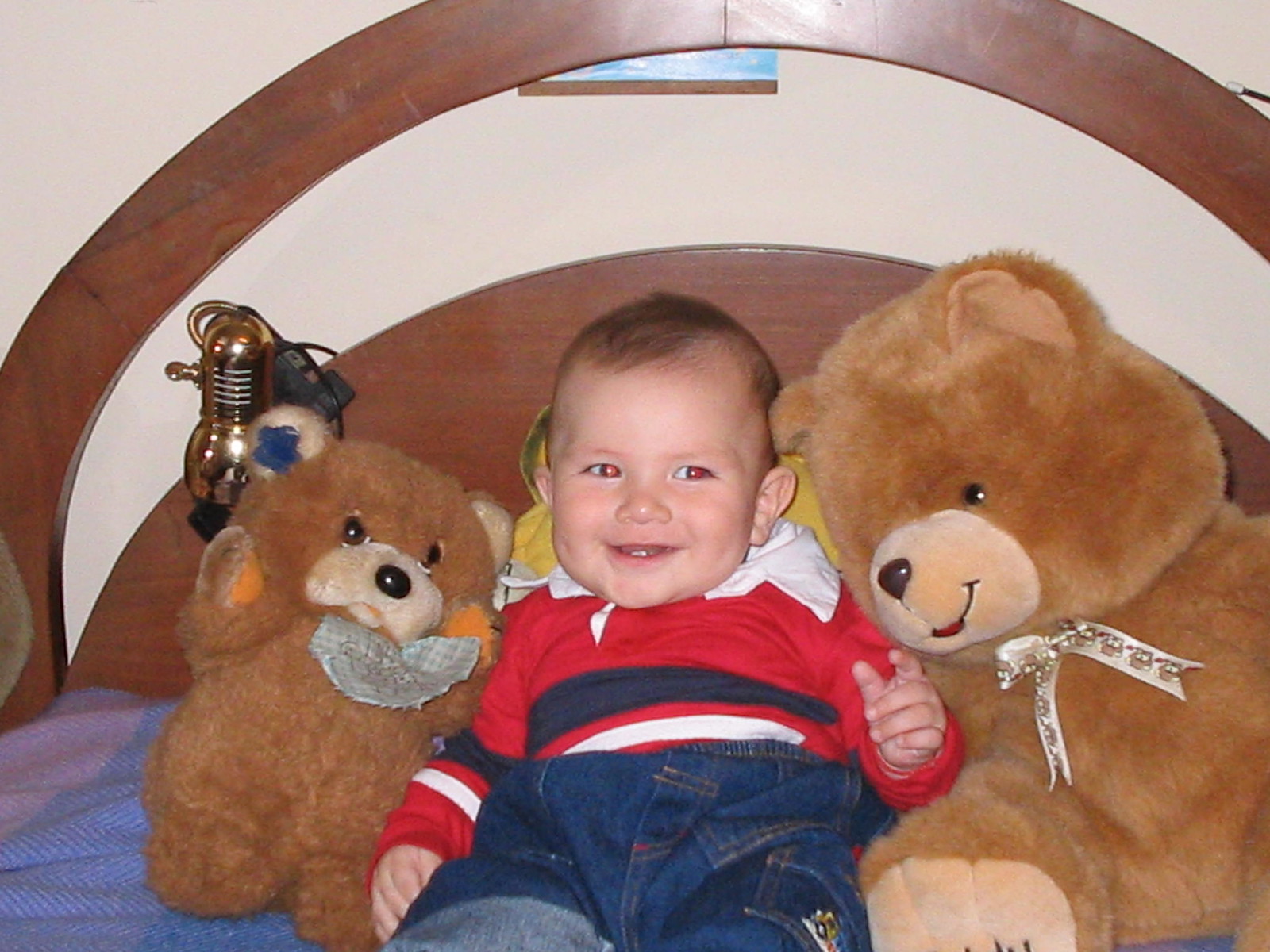The image captures a smiling baby or toddler, likely between four to six months old, lying on a bed with light blue sheets. The infant has thin brown hair, prominent ears, and is dressed in blue jeans and a red long-sleeved shirt featuring blue and white stripes along with a white collar. Each side of the baby is flanked by a brown teddy bear; the larger bear, on the baby's right, wears a ribbon tied in a bow around its neck, while the smaller bear on the left is adorned with a bib. The wooden headboard, which features a crescent moon cutout, and a white wall serve as the background. Additionally, there is a small gold lamp or microphone fixture visible near the headboard, potentially attached to it by an electrical cable. The baby is looking and smiling to the left, appearing joyful and engaged with whoever is capturing the moment.